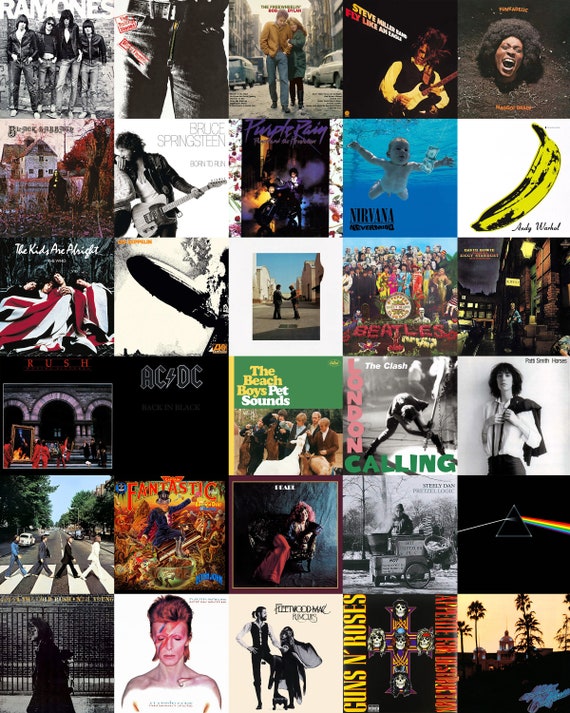This detailed collage consists of 30 uniformly sized squares, each featuring album covers from a variety of iconic bands and artists spanning multiple genres. The top left starts with The Ramones, followed by an indiscernible jeans image, and then a man and woman walking down the street. Additional covers depict The Steve Miller Band, a woman with an afro, and Black Sabbath featuring Ozzy Osbourne in front of a white house and tree. The collection includes Bruce Springsteen's 'Born to Run', Prince's 'Purple Rain' with him on a motorcycle enveloped in purple haze, and Nirvana’s 'Nevermind' featuring a swimming baby chasing a dollar bill. Andy Warhol’s banana artwork appears, followed by The Who's 'The Kids Are Alright'. 

Positioned in the rows below, you find Rush members sleeping beneath a British flag, Led Zeppelin’s image of the Hindenburg crash, and a scene of two people shaking hands. There’s also The Beatles surrounded by flowers with fans in the background. Nearby is a musician seemingly arising from a building with an indistinct title. Other notable covers include ACDC, The Beach Boys’ 'Pet Sounds', London Calling by The Clash, and Patti Smith. Further down are The Beatles walking on a street, an image of a man in a black suit on a bullet, a daybed scene with a woman in black pants and pink hair, Steely Dan fronting a pretzel cart, and Pink Floyd's prism with a rainbow. The lower row features David Bowie with a lightning bolt on his face, Fleetwood Mac, Guns N' Roses, and an architectural scene that resembles a church in Florida.

This vibrant, genre-crossing montage unites legendary album art from artists like Guns N' Roses, Fleetwood Mac, David Bowie, The Beatles, The Beach Boys, Pink Floyd, AC/DC, Rush, and Led Zeppelin, showcasing a compelling visual history of influential music and culture.